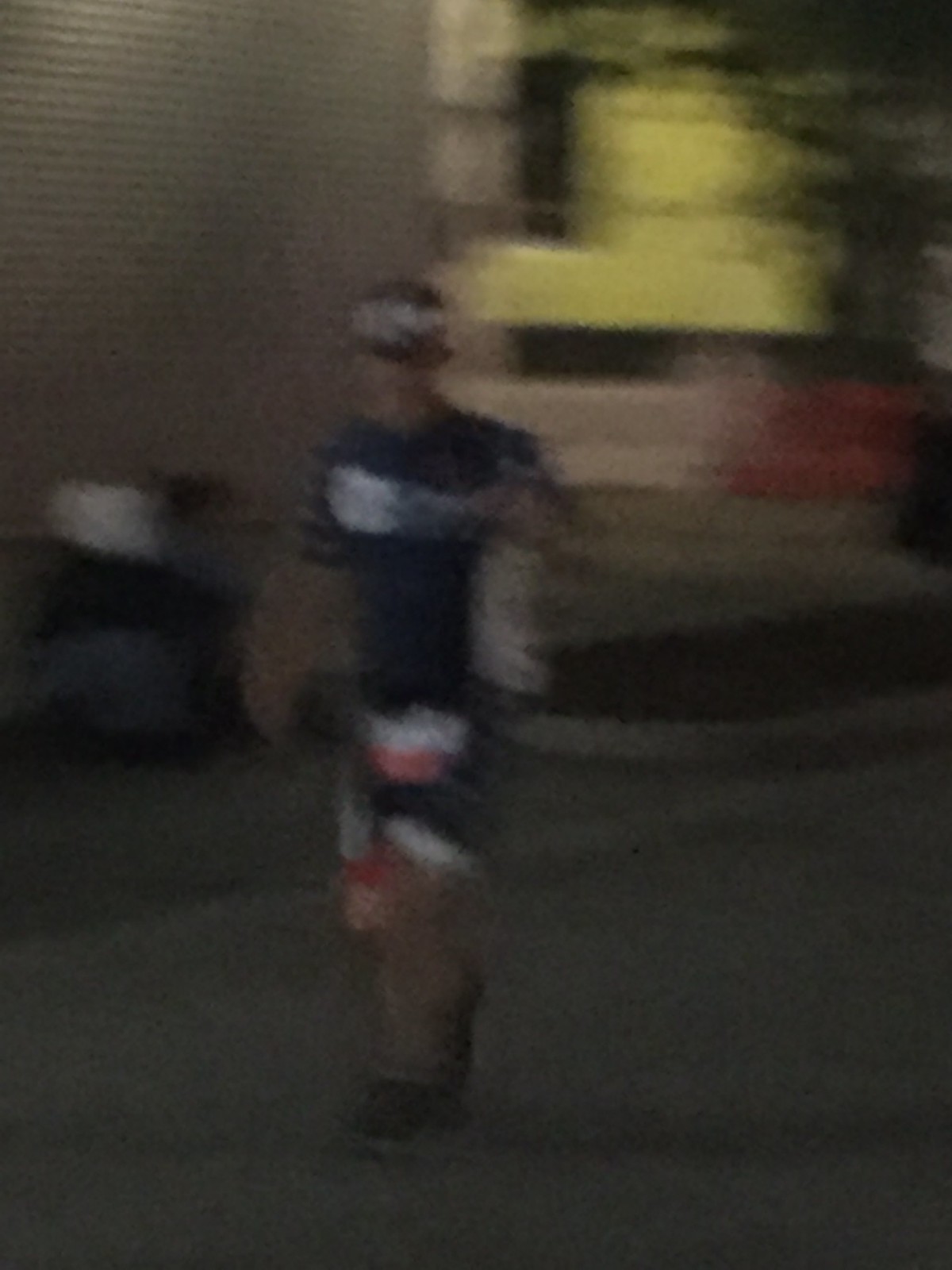In the very blurry and dark image, a man resembling a construction worker or possibly a marathon runner is captured walking or running down a street. The man appears to be wearing a black or blue shirt with some white lettering across the chest and may have a long-sleeved brown shirt underneath. He sports a helmet or cap with potential stickers or writing, hinting at construction work. He also has shorts that feature colors such as white, red, black, and possibly orange, with brown pants or something wrapped around his waist hanging down. The man's legs are in motion, adding to the blur, and he may be wearing boots or sneakers. The setting includes a large red-brick building behind him, another structure with yellow parts to the right, and a car visible in the background. The photo's graininess and darkness obscure further details, making it challenging to discern specific elements clearly.